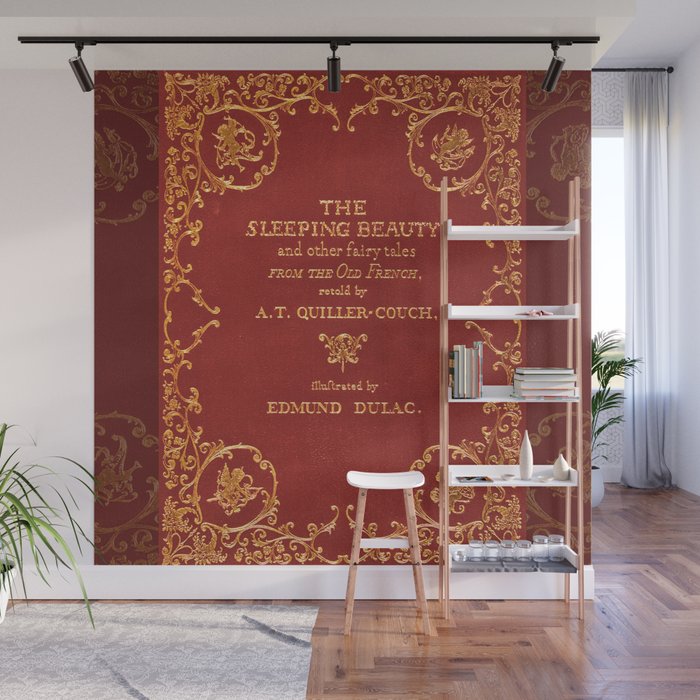This photograph captures a cozy room in a house featuring a striking wall transformed into a giant reproduction of an old-fashioned leather-covered book, with elaborate gold engravings on a red background. Prominently displayed in gold and silver lettering, the book cover reads: "The Sleeping Beauty and Other Fairy Tales from the Old French, retold by A.T. Quiller-Couch, illustrated by Edmund Dulac." This unique wall separates two rooms in the house. Above it, a black strip running across the ceiling houses three black lights illuminating the faux book cover.

In front of this imaginative wall is a five-shelf wooden unit with white shelves. The shelves hold various items including books, small sculptures, and a row of clear glass votive candles on the bottom shelf. Positioned almost centrally against the book cover, the shelf stands alongside a white stool with light brown wooden legs. The room features a wooden parquet floor, partially covered by a rug on the left. Adding to the décor, two potted plants are strategically placed—one to the left of the shelf and another to the right, near a window. This window, adorned with white drapes, allows natural light to flood into the room, enhancing its welcoming ambiance.